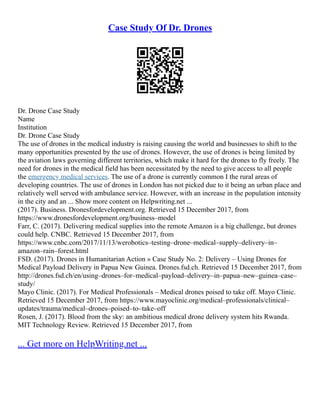The image shows a detailed document titled "Case Study of Dr. Drones" in prominent blue letters at the top. Directly below this title, a black and white QR code features three dots at its top, right, and bottom corners, designed for scanning. The document is densely filled with black text, including many empty spaces for users to fill in personal information such as name and location. The body of the document consists of two to three short paragraphs, written in small, neatly arranged lines. At the bottom, in blue text, the phrase "get more on healthwriting.net" is followed by a blue line stretching across the page.